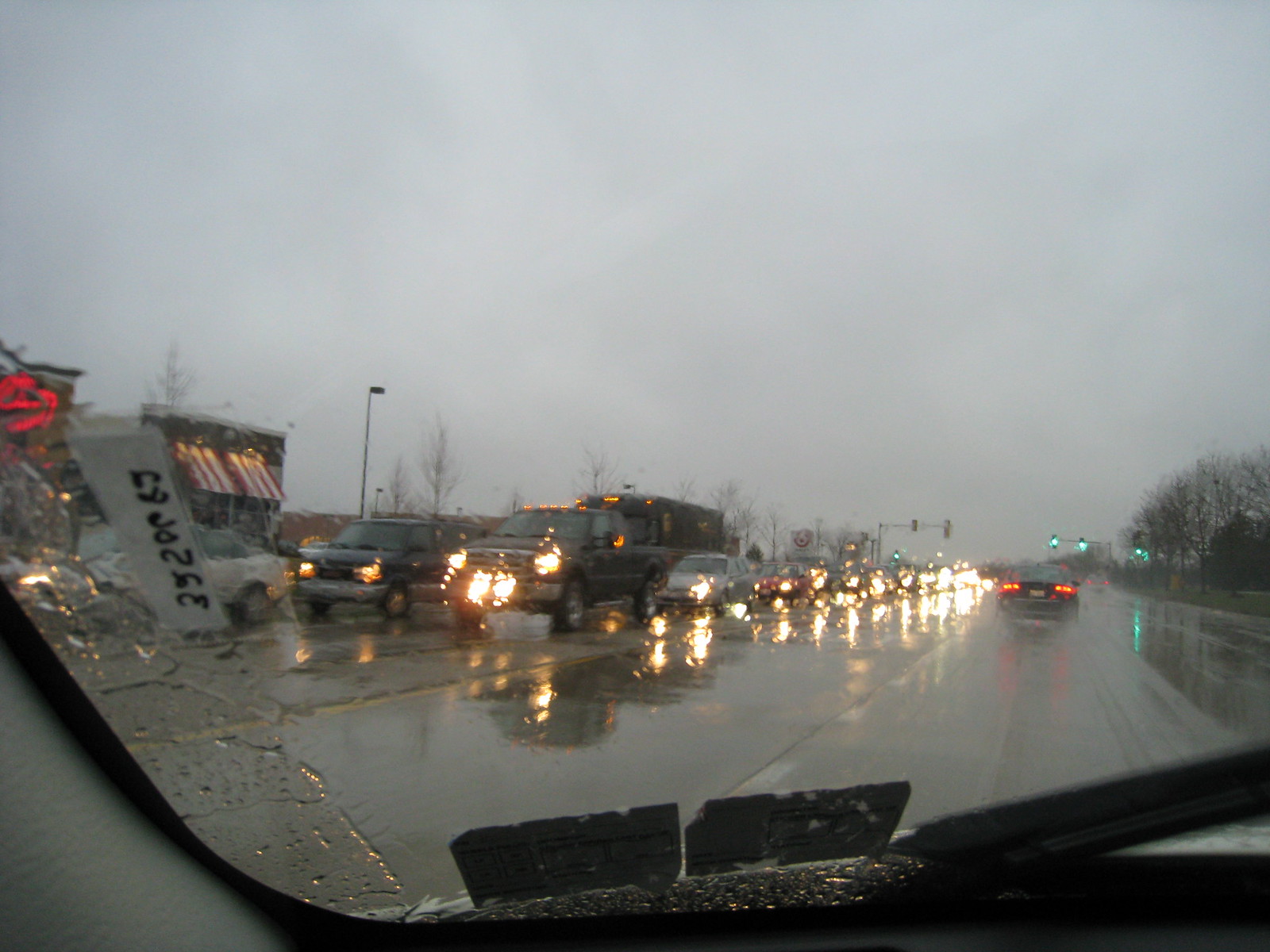This color photograph, taken from inside a car through a rain-streaked windshield, captures a dreary roadside scene during a storm. The sky is completely overcast with dark, gray clouds, casting a dim light over the wet, reflective road. The image shows a two-lane roadway, with heavy traffic on the left side going in the opposite direction, all vehicles with their headlights on, creating a shimmering reflection on the rain-soaked street. The right side, where the car is traveling, has minimal traffic with only one vehicle ahead. Water droplets blur the lights of the oncoming traffic. To the left, buildings with various signs are visible, including a distinct red and white awning and what appears to be a Target sign further back. The scene is framed by a few lifeless-looking trees on the right, adding to the gloomy atmosphere. Inside the car, the corner of the windshield wiper and a couple of stickers on the windshield are visible, providing context to the viewer's perspective.